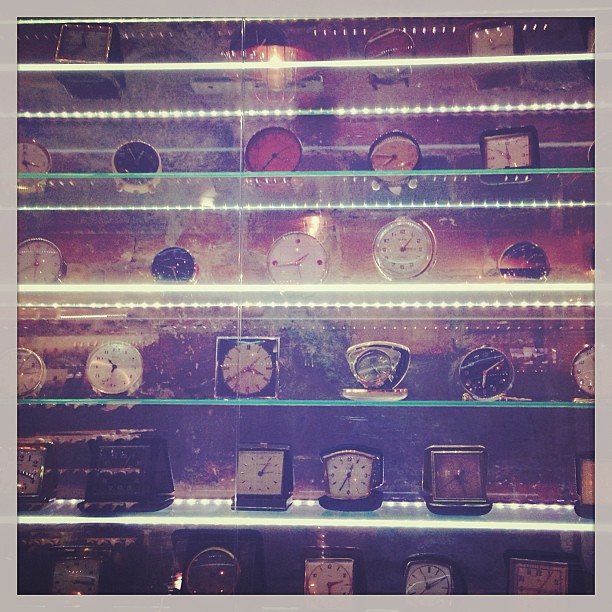The image depicts an elaborate display of various clocks arranged on multiple glass shelves. The shelves extend vertically to the top of the frame, allowing a view of the clocks from underneath. The collection includes circular and boxy-shaped clocks in a range of colors such as red, white, gray, and black. Many of the clocks feature intricate, expensive-looking designs with golden trims. Each shelf is illuminated by a line of white lights positioned at the back, enhancing the overall visibility and aesthetic appeal of the display. The background features a detailed illustration with a gradient from darker green at the bottom to lighter hues of white and red towards the top.